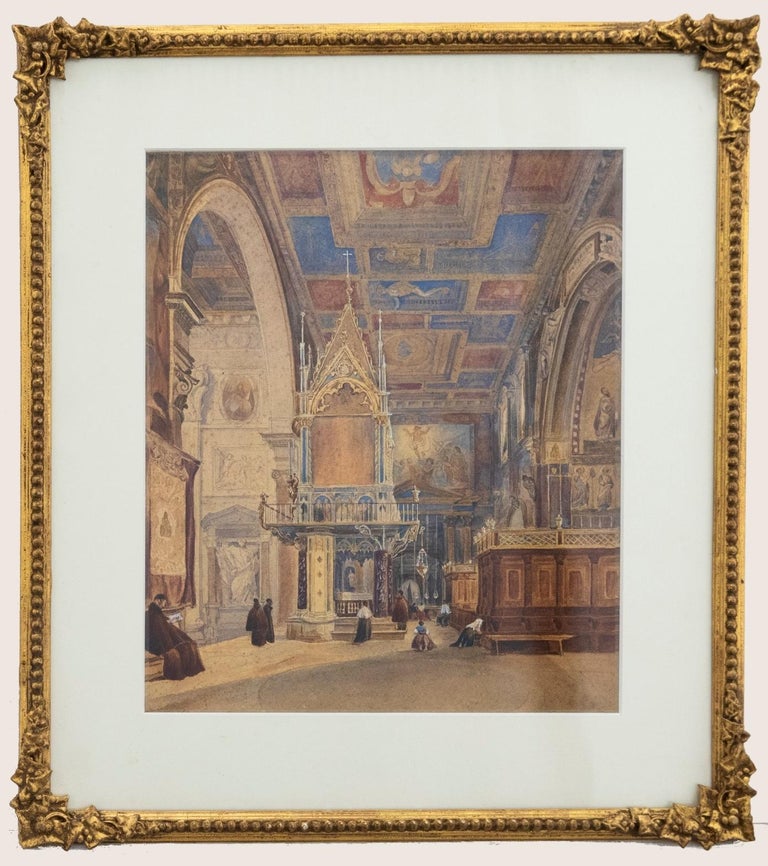This detailed photograph showcases a framed Renaissance painting, encased in an ornate golden frame adorned with decorative leaves, flowers, and rounded dots along its edges. The artwork vividly depicts the grand interior of a monumental building, possibly the Sistine Chapel, with its immense archways and intricately painted ceilings. The walls and ceilings are adorned with various murals, although they appear somewhat faded over time, making individual details hard to discern. The scene bustles with figures, including several in monk robes; one notable character is positioned toward the left with short black hair. Other distinctive figures include a person in a white shirt and baggy dark pants, one in a blue shirt with white sleeves and brown pants sitting to the right, and religious figures dispersed throughout the space. The painting, ensconced in its golden frame, hangs on a white wall, offering a window into a historic and architecturally significant moment.